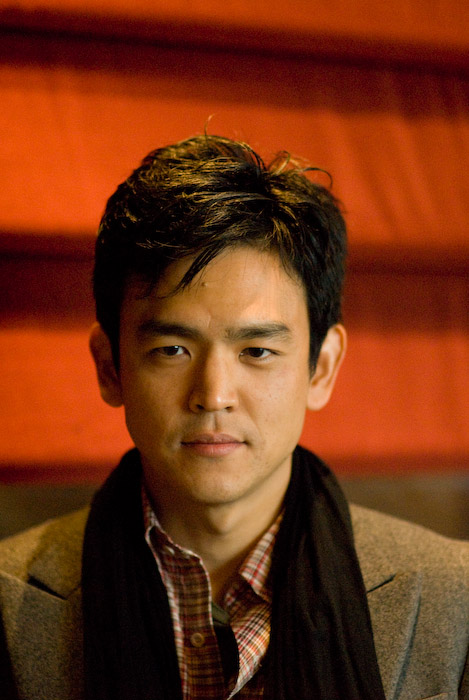In the image, famed actor John Cho, renowned for his roles in the "Harold & Kumar" films and the "Star Trek" series, is depicted wearing a stylish ensemble consisting of a black suit complemented by a black scarf and a red flannel shirt. His slightly tousled hair drapes over one of his sharply defined eyebrows, adding an element of casual allure to his look. Cho gazes slightly to the left, his expression contemplative, with his nose subtly inclined downward. The backdrop features a warm gradient of orange transitioning into a gray layer, providing a striking contrast that enhances the profile nature of the shot. His poised demeanor and detailed attire capture both elegance and a hint of rugged charm.